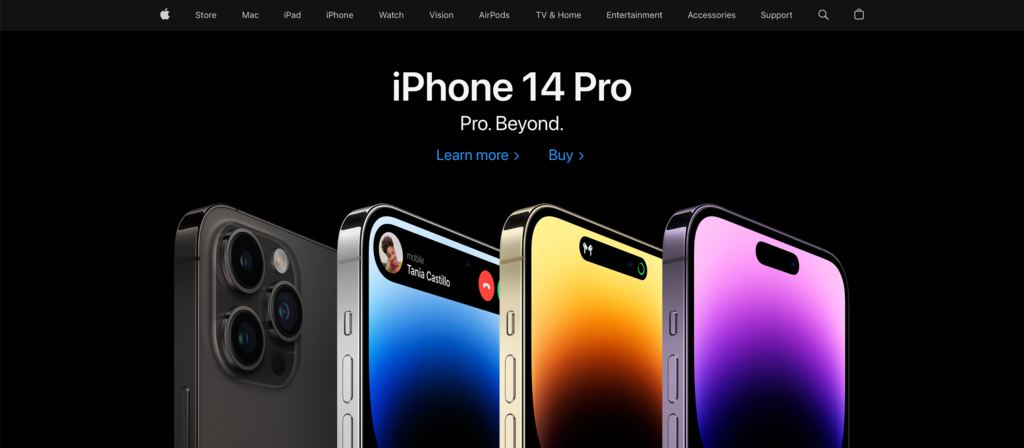The image appears to be a screenshot of the Apple website, likely showcasing the latest iPhone model. At the top, a thin dark gray banner stretches across the page, featuring the Apple logo followed by a series of menu options in small font: Store, Music, iPad, iPhone, Watch, Vision, AirPods, TV & Home, Entertainment, Accessories, and Support. A search icon in the form of a magnifying glass is also present.

Directly below the banner, against a black background, large white text announces "iPhone 14 Pro." Beneath this, the tagline "Pro. Beyond." is displayed, with each word followed by a period. Further down, two blue buttons offer additional options: "Learn more" with an arrow pointing right, and "Buy" with an arrow pointing right.

Central to the image are four iPhones partially visible from top down, arranged from left to right. The first iPhone, on the far left, is gray and displays its back with three camera lenses and a flash. The next three iPhones show their front screens - one silver with a blue screensaver, one gold with a gold screensaver, and one light purple with a purple screensaver.